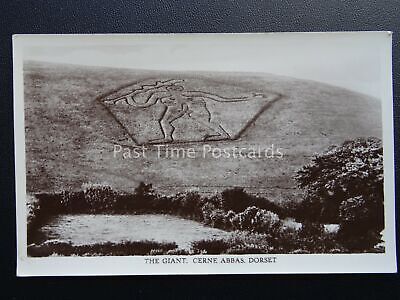The image depicts a black and white postcard, which is affixed to a dark, textured background, possibly a wall or a stand. The postcard is labeled in white text with a watermark in the center reading "past-time postcards." The scene on the postcard shows an outdoor landscape with a central feature: a large drawing on a mountainside or hill, illustrating a naked man holding what appears to be a rod of lightning. This figure is outlined prominently against a natural backdrop of trees, and there may be water, such as a pond, among the trees. The bottom of the postcard is captioned with the text "The Giant CERN ABBAS Dorset," referring to the location and the name of the ancient figure depicted. The overall image quality is low, but the details are discernible, highlighting the mysterious and intriguing nature of the scene.